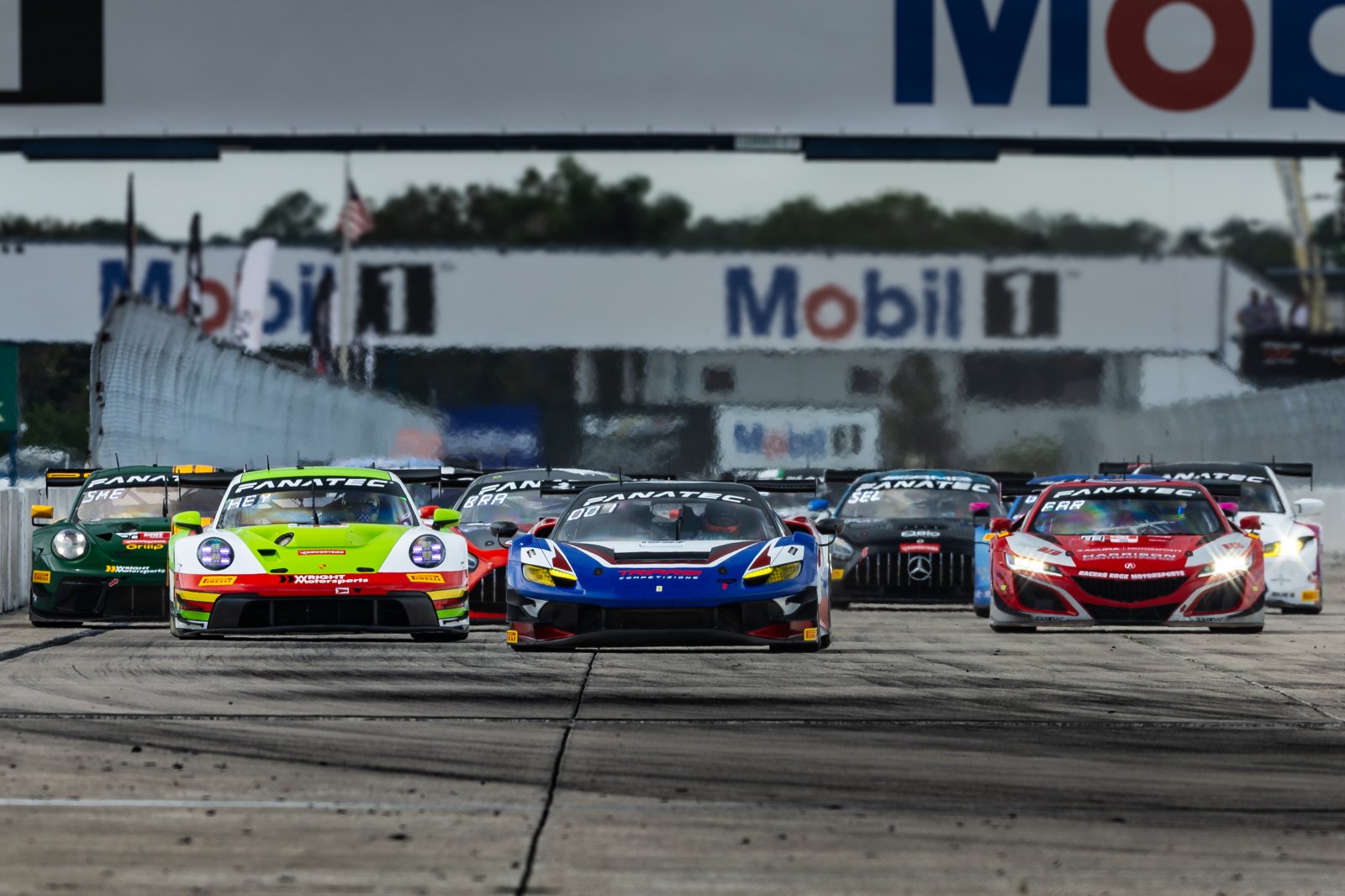The photograph captures a high-energy moment of cars racing on a racetrack, with a clear emphasis on branding and details of the vehicles. The image features a brightly lit racetrack with Mobil 1 sponsorship prominently displayed on multiple billboards and banners, including a white overhead sign with the Mobil 1 logo, where the "O" is distinctively red and the other letters are blue.

In the front row, three cars are positioned side by side: the car on the far left is lime green and white with a red bumper, the middle car is blue with a black and white hood, and the car to the far right is red with some silver accents. Behind them, in the second row, a dark green car can be seen on the far left, next to a car that appears gray but is partially obscured by the blue car in the first row. Next to this is a light blue car with a prominent Mercedes-Benz grille and emblem, followed by a white car.

All the cars display the word "Fanatec" along the top of their windshields, hinting at a possible racing team or brand affiliation. The background is set in a natural environment with trees and greenery, adding contrast to the contemporary race scene. Both the vibrant colors of the cars and the detailed track setting contribute to a realistic and immersive depiction of the race.